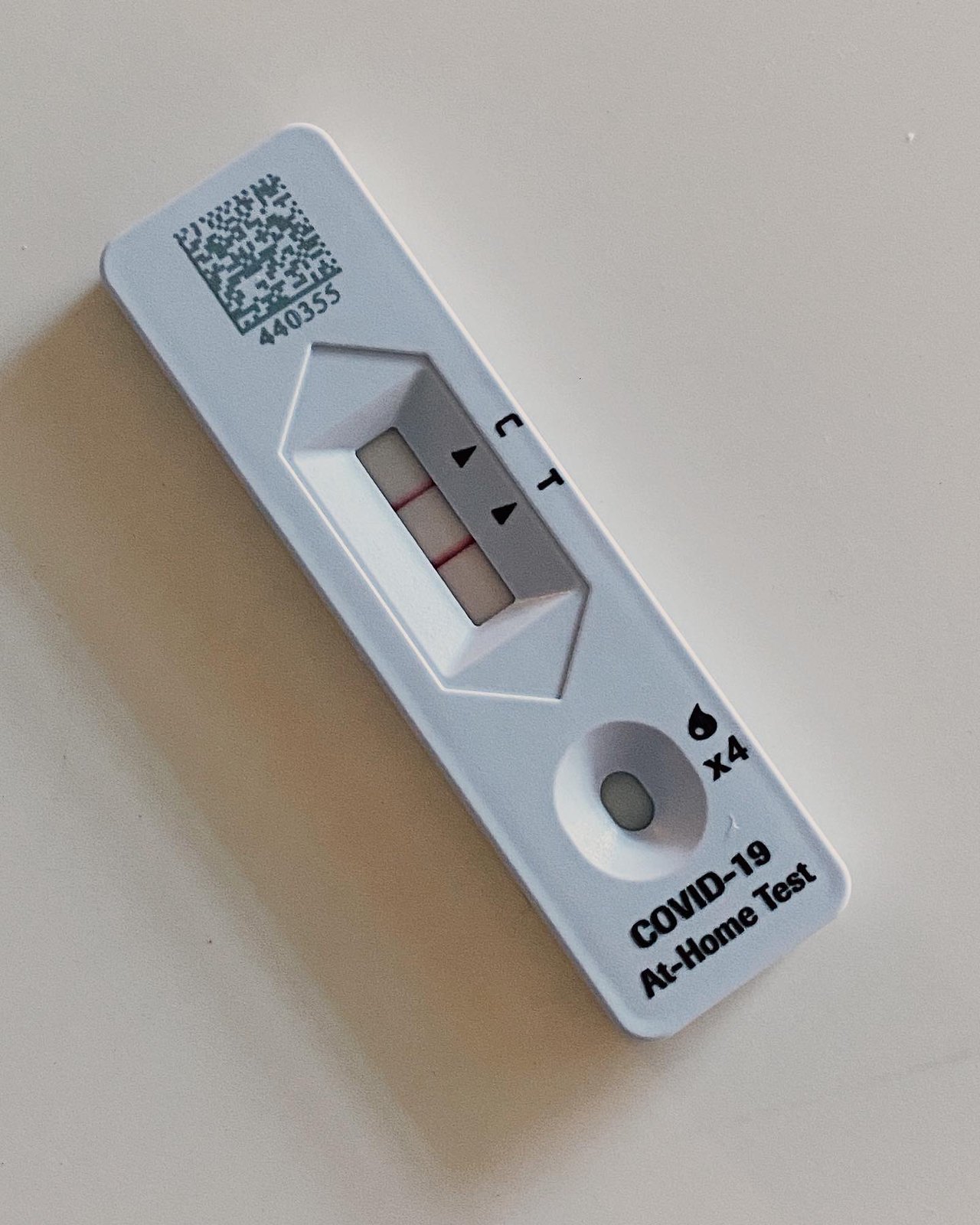In this detailed image, a COVID-19 at-home test is prominently displayed on an off-white countertop. The test, rectangular in shape, features a clear black text label at the bottom identifying it as a COVID-19 test. 

At the top of the test, there is a QR code marked with the numbers "440355," which can be scanned for additional information or verification. Below the QR code, the test area prominently displays a diamond-shaped window where the results are shown. This particular test window reveals two red lines, signifying a positive result. The first red line, towards the top of the diamond shape, corresponds to the control (C) line, while the second red line, below the first, indicates the test (T) line.

Directly beneath the diamond-shaped result window is a small, circular sample well where the collected sample is to be placed. To the right of this sample well, there is a water drop symbol accompanied by "×4," instructing the user to add exactly four drops of the sample to ensure accurate results.

The image also captures a subtle shadow cast by the test, slightly extending to the left, adding a bit of depth to the photograph.